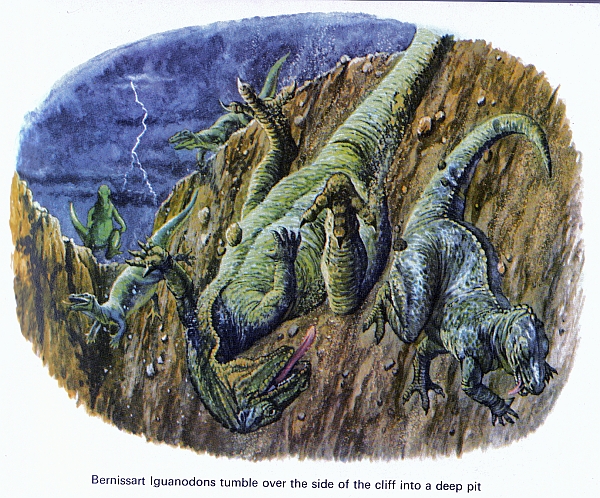The illustration vividly depicts a dramatic scene where several green dinosaurs, including what appears to be T-Rexes and iguanodons, are tumbling off a cliffside amidst a thunderstorm. The sky is a dark, ominous blue, split by a striking bolt of lightning. The rocky cliff from which the dinosaurs fall is primarily brown with splashes of orange and green. One dinosaur, its tongue lolling out in apparent fear, is prominently shown diving head-first down the cliff. Accompanying this creature, two others are also in free fall, positioned head-down, seemingly doomed to follow their peer into the abyss. Meanwhile, at the edge and corner of the cliff, other dinosaurs look down, almost mockingly, at their falling companions. Scattered gray and brown rocks accompany the dinosaurs in their descent. At the bottom, the label reads in black sans serif font, "Vernisart iguanodons tumble over the side of the cliff into a deep pit," adding a final note to this vividly chaotic scene.